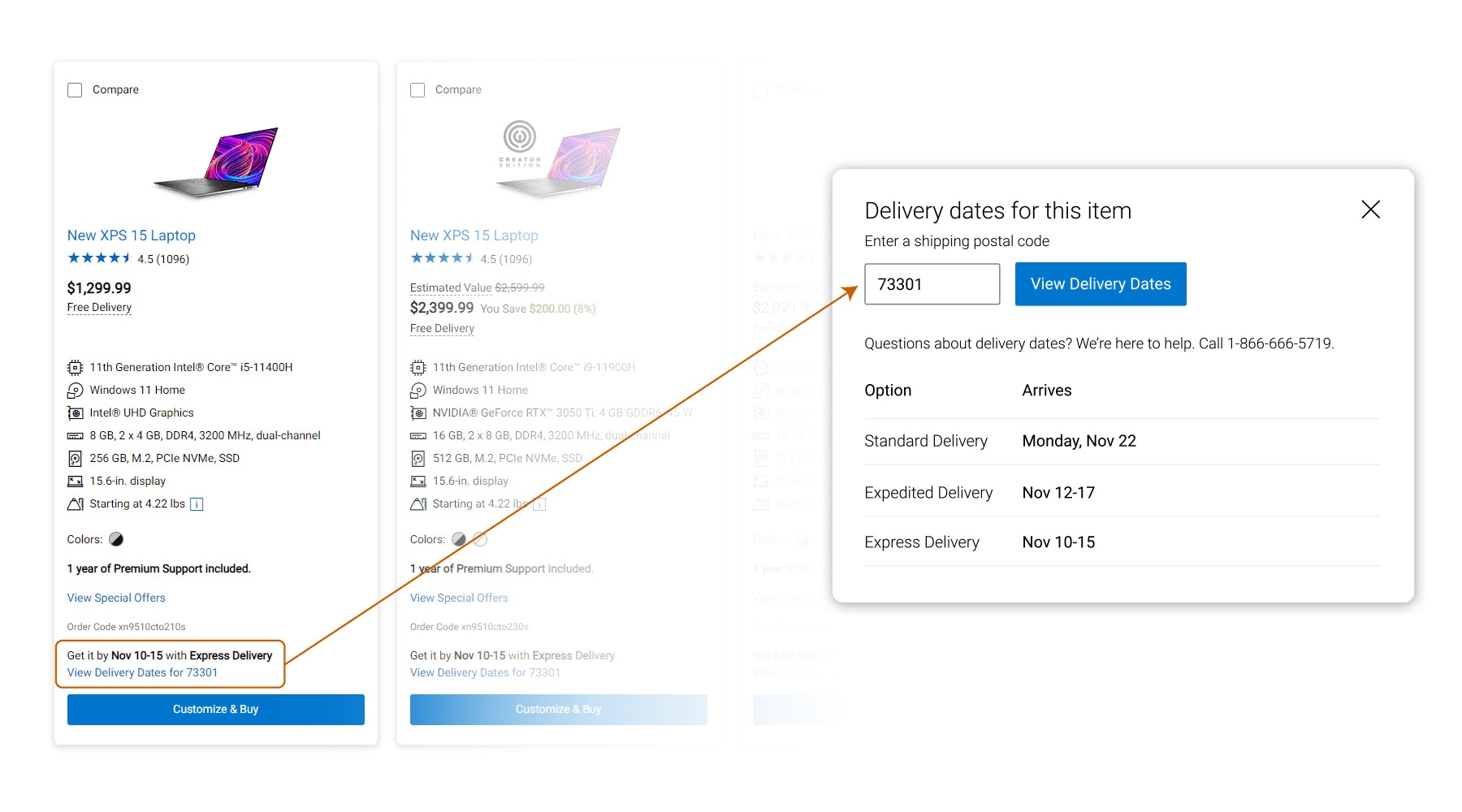On the far left side of the image, there is a long box displaying a laptop. The laptop screen features various shades of purple. Beneath the laptop image, the text reads "New XPS 1.5 Laptop" followed by a rating of four and a half out of five stars. The price, displayed in black text, is $1,299.99, and it also mentions free delivery. Below, there is an outlined box in orange that states, "Get it by November 13th through 15th with express delivery."

A long line extends from this orange box to a box on the right side, pointing to the postal code "373301." Adjacent to this, the text in blue reads, "View delivery dates." The delivery options are listed as follows: standard delivery arriving on Monday, November 22nd; expedited delivery between November 12th and 17th; and express delivery between November 10th and 15th.

Returning to the left side, directly beneath the orange outlined box, there is a blue box with the option to "Confirm and Buy." Above the orange box, in black text, it states, "One year of premium support included."